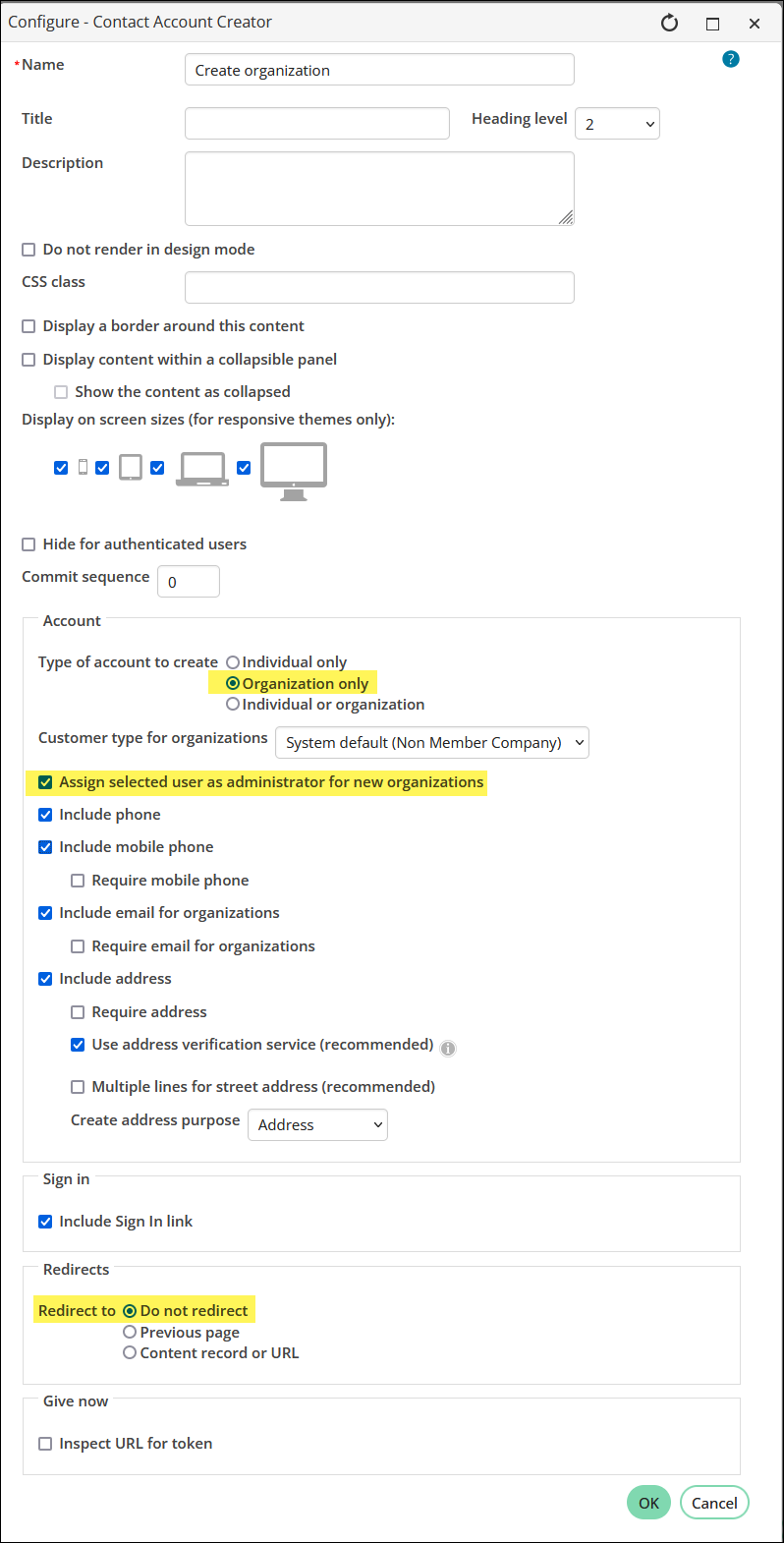The image portrays a website interface featuring a detailed configuration form for creating an iPart contact account. The form is titled "Create Organization" and is marked as a heading level 2. Key elements include:

- A text field labeled "Name" with a mandatory red asterisk.
- Options to display a border around the content and to display content within a collapsible panel.
- Choices for showing the content as collapsible and for responsive display across various devices, represented graphically from a small iPhone to a desktop computer. Each device icon has a checkbox on its left, all marked in blue and checked in white.
- Additional options like "Hide for authenticated users," "Commit sequence under account," and "Type of account to create (individual or organization)," all checked off in green.
- Features for assigning the selected user as an administrator for new organizations, and options to include iPhone, mobile phone, and email for organizations, each checked in blue. However, "Require email for organizations" is not checked.
- Further settings include "Include address," "Use address verification," and "Redirect to" with a "Do not redirect" option highlighted in yellow.

Overall, the image meticulously details a complex form for configuring various attributes and settings of an organization account within a web-based interface.